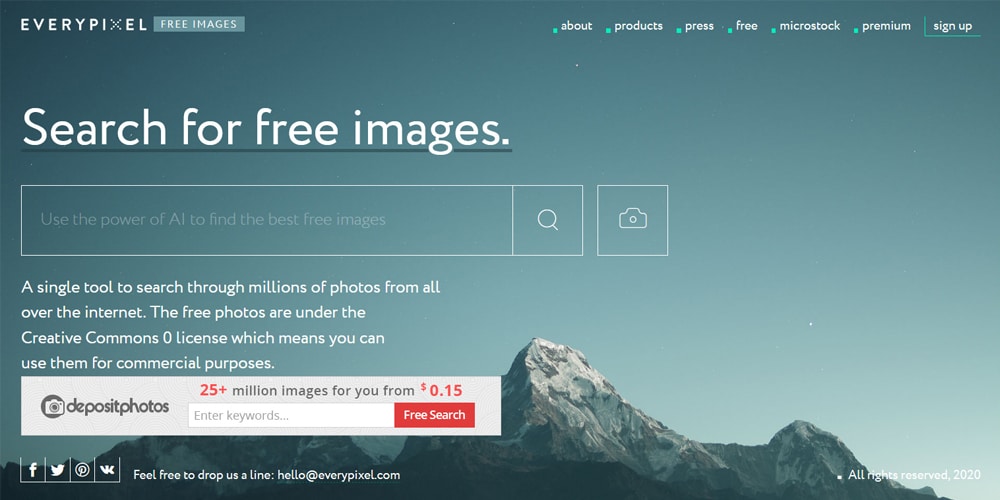This is a detailed and cleaned-up caption for the described image:

---

This rectangular landscape image, akin to the shape of a laptop screen but slightly wider, depicts the interface of an image search website. The ratio of its width to height is a bit more than 2:1. The background features a light blue sky transitioning to a darker blue-green hue towards the top left, with Rocky Mountains along the bottom. The image appears to be an illustration rather than a photograph.

In the upper left corner, the company's logo, "EveryPixel," is displayed in white text within a dark blue-green box. The "X" in "EveryPixel" is pixelated, which is part of their branding. Adjacent to the right in a lighter blue box, "FREE IMAGES" is boldly written in uppercase white text.

From the center to the right edge of the image, there are seven selectable areas. The first six feature bright aqua circles with white lowercase text to their right, each representing different sections: "products," "press," "free," "microstock," "premium," and "sign up." The "sign up" selection differs in that it has a rectangular outline with the same aqua color but only shows the bottom and left sides of the box.

The background lightens to a teal-tinted sky towards the middle. Prominently in the top-left area, in large white font with a dark blue-green underline, is the text "Search for free images." Below this, a large, clear search box maintains the background view, outlined in thin white. Inside, faint white text reads, "Use the power of AI to find the best free images," accompanied by a magnifying glass icon. To the right of the search box is a separate square with a camera icon for video searches.

Beneath the search box, aligned left, are four lines of small, bold white text, double spaced for clarity. They state: "A single tool to search through millions of photos from all over the Internet. The photos are under the Creative Commons zero license, which means you can use them for commercial purposes."

A long, light green rectangular box lies below, matching the search box's size. On the left in dark gray, it says "depositphotos," preceded by a camera icon. To the right, there's another search field, possibly for a different company's search function.

At the bottom, the left corner hosts standard social media icons (Facebook, Twitter, Pinterest, and TikTok) with accompanying text. The right corner also contains small white text.